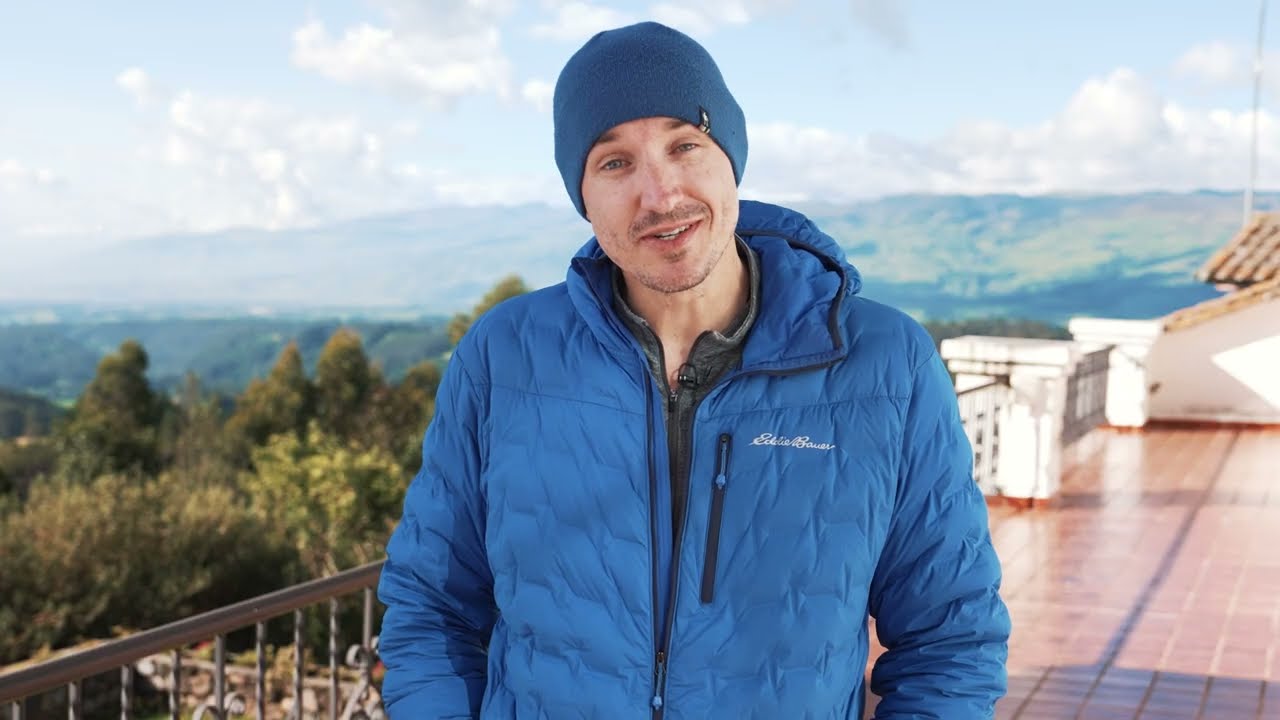A man in his late 20s or early 30s stands on a balcony, potentially the rooftop platform of a building, overlooking a scenic valley. He's wearing a medium blue winter jacket, partially zipped up with a gray shirt peeking from underneath, and a matching tight-fitting blue cap. His hands are in his pockets, and his head is slightly tilted to the right, with his mouth partially open as if he's speaking, possibly as part of a podcast or instructional video. To the left, the balcony's railing frames some trees below, and to the right, white rooftop tiles extend into the distance. The background features partially cloudy skies with patches of blue, and towering green hills or mountains. The overall color palette of the image includes blues, whites, and greens, giving a sense of a cold, late winter or early spring day.